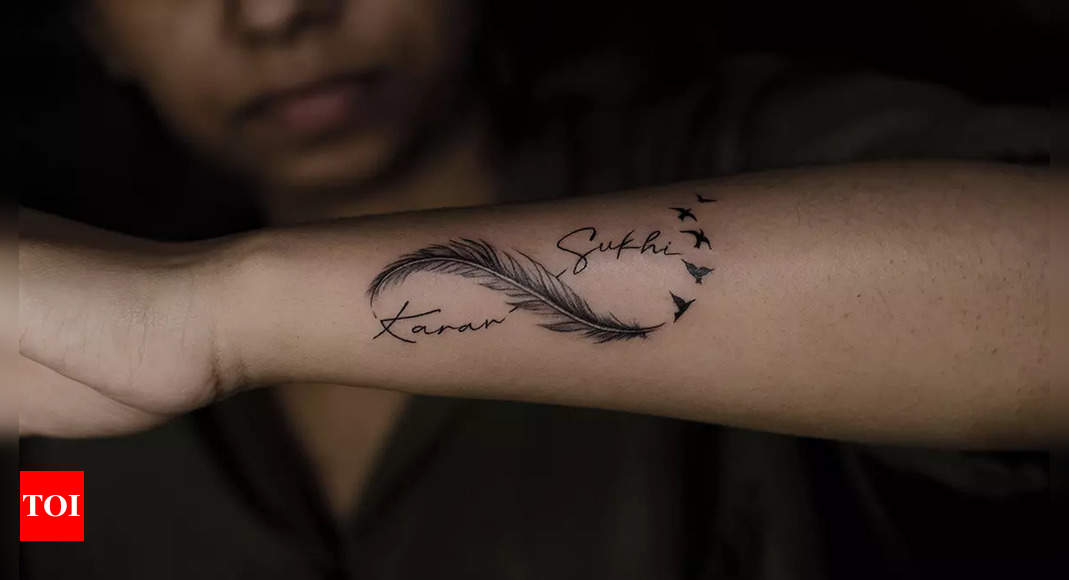The photograph captures a detailed image of a girl's left forearm, prominently displaying a finely detailed tattoo on the outer side, between her wrist and elbow. The intricate tattoo features a stylized figure-eight design, which is creatively composed of a feather that morphs into a series of birds flying away. The feather design flows gracefully in a wave-like fashion, with the birds delicately trailing off from its tail. Within the tattoo, two names, "KARAN" and "SUKHI," are inscribed in a cursive script, each name positioned on either side of the figure-eight. The tattoo is rendered in black ink, highlighting the meticulous line work and fine detailing. The girl's partial face is visible, blurred out from the nose down, against a slightly darker skin tone background. A small red square with the white capital letters "TOI" in the bottom left corner suggests that this might be a portfolio shot showcasing the tattoo artist's delicate and intricate work.